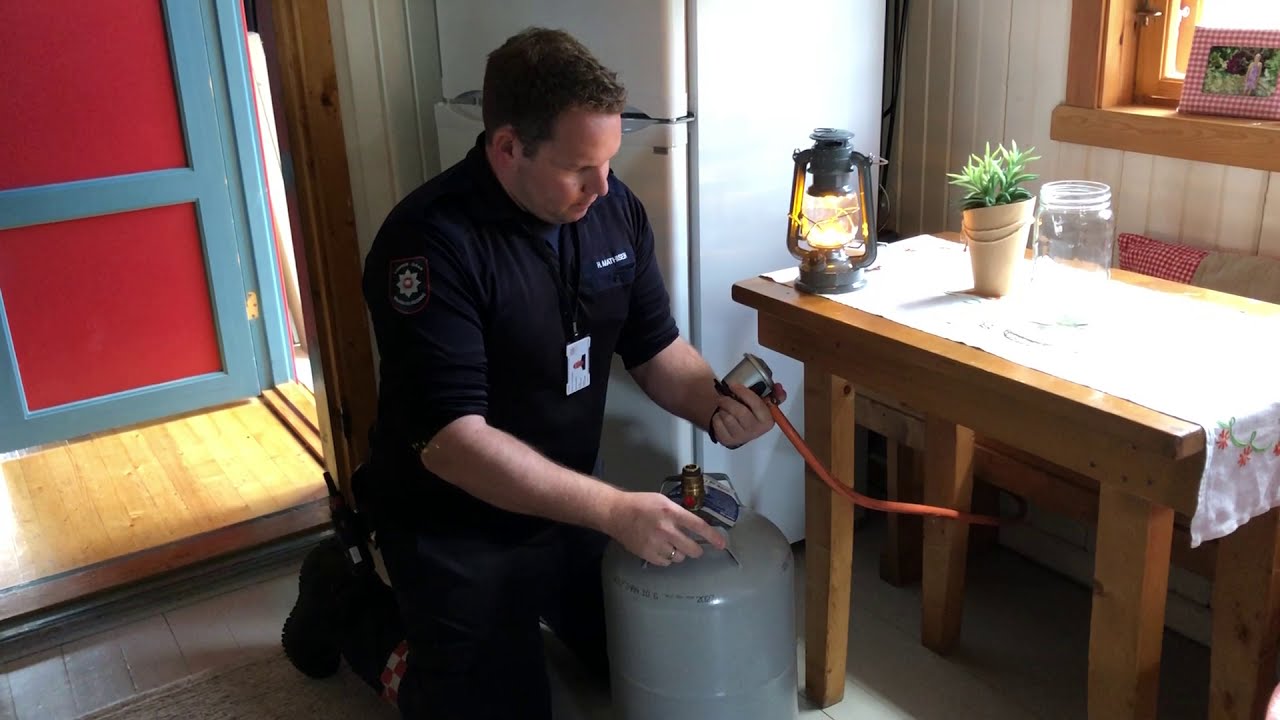In the rural indoor kitchen, a Caucasian man with light brown hair kneels beside a gray propane tank. Dressed in a dark blue uniform with a star on his right shoulder and an ID badge hanging from a lanyard around his neck, he carefully attaches a silver, cup-like valve with an orange tube leading away from it to the tank. The uniform, which has long sleeves pulled up to the elbows, suggests he might be a service or government official. A walkie-talkie hangs from his belt, and he wears black shoes.

Next to him is a wooden table covered with a white tablecloth, upon which sits a lit, gray kerosene lamp casting a soft yellow light. The table also features a small light brown cup with a green plant and an empty glass jar. Behind the man is a white refrigerator, and to his right is a door with a blue frame and red panels that stands open, allowing light to spill onto the yellow, slatted-panel floor. A framed photo with a red plaid border is perched on the window ledge above the table, completing the rustic, cozy kitchen setting.